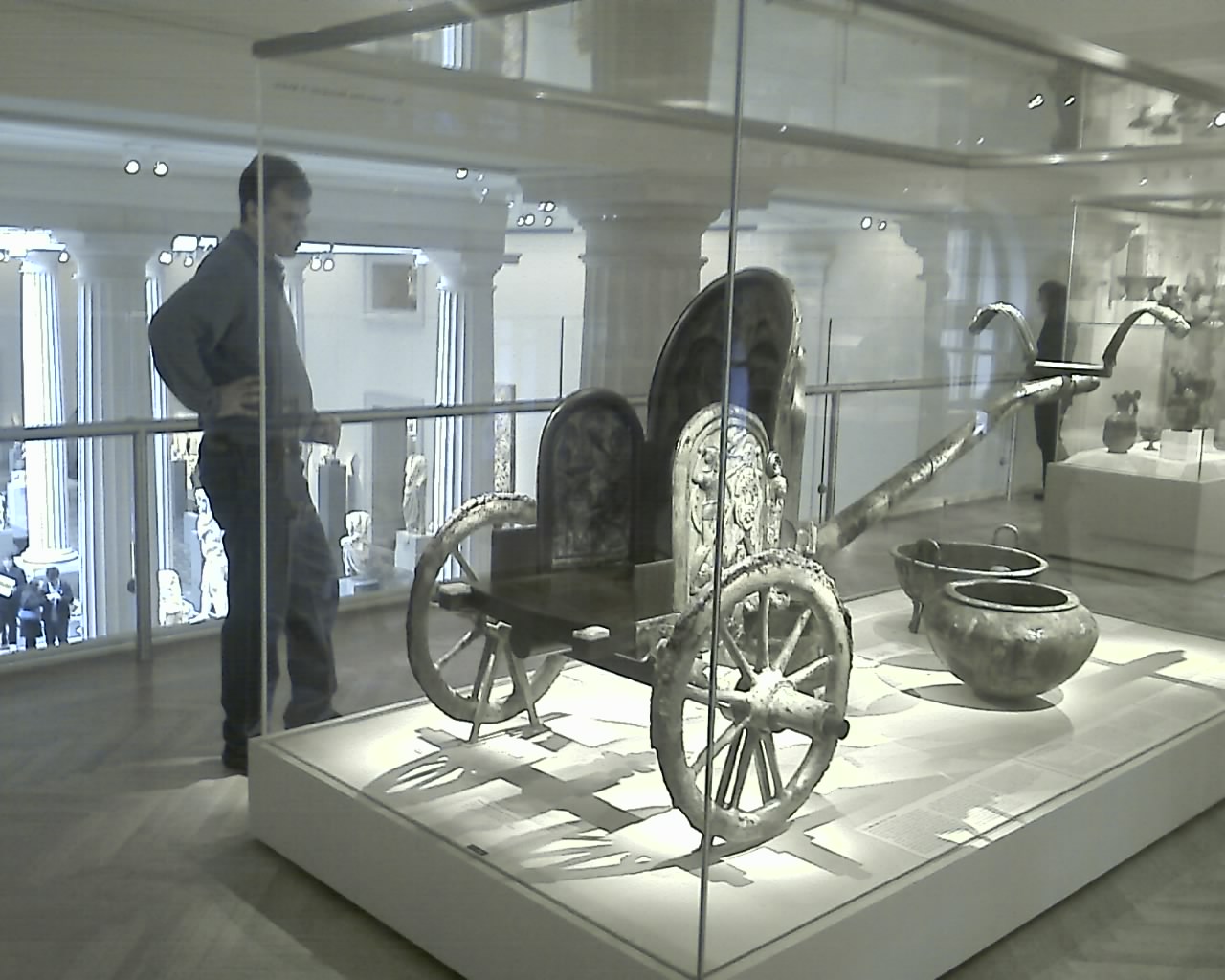The photograph depicts a brightly lit museum interior showcasing an ancient, two-wheeled carriage-like artifact, likely of Roman or Greek origin. This intricately crafted vehicle, meant for a single person to stand in, is enclosed in a clear glass case. It's positioned in a spacious, predominantly white space with numerous white columns and statues, alongside other antiquities. A man, dressed in dark clothing and showcasing a distinct posture with his hand on his hip, stands near the glass case, intently observing the artifact. The museum features a second-floor layout, offering a view of additional displays and antiquities on the lower level through large windows. The overall ambiance is one of modern minimalism, with white and silver tones dominating the scene.